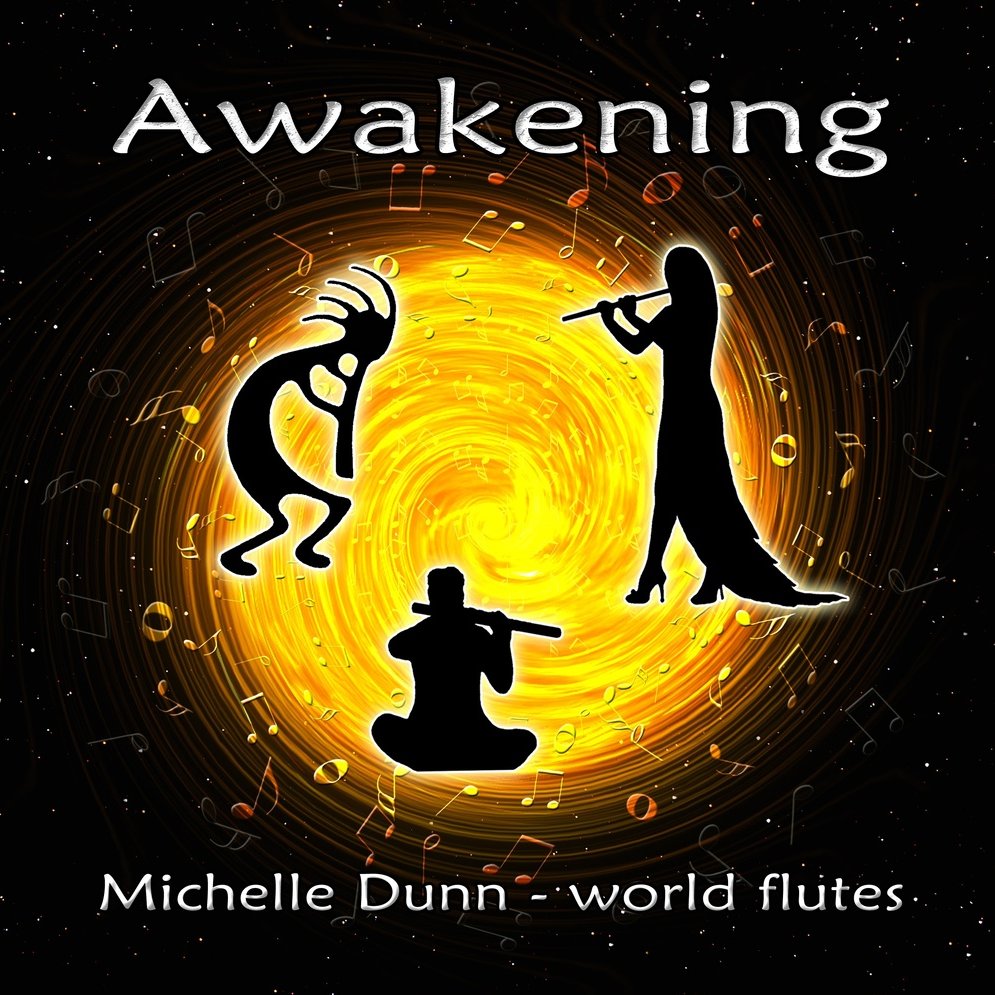The image, resembling an advertisement or an informative poster, features a vibrant, fiery spiral at its center, set against a backdrop of a black night sky filled with stars. The spiral, reminiscent of a tornado, showcases a blend of warm colors including yellow, orange, and red. At the top of the image, bold text reads "Awakening," and at the bottom, it says "Michelle Dunn - World Flutes."

Within the swirling, flame-like spiral are three black silhouettes positioned in a triangular formation. On the left, a mystical creature-like figure bends over, playing a flute. On the right, a female figure, possibly with a tail, stands in profile, also playing a flute. At the bottom, a male figure sits with his back to the viewer, immersed in playing a flute.

Musical notes abound within the spiral, adding to the dynamic and magical ambiance of the scene, which is further emphasized by the starry expanse beyond. The overall design is highly stylized, illustrating a fusion of surrealism and musical themes, likely intended to capture the viewer's imagination and highlight the thematic elements of "Awakening" and "Michelle Dunn - World Flutes."